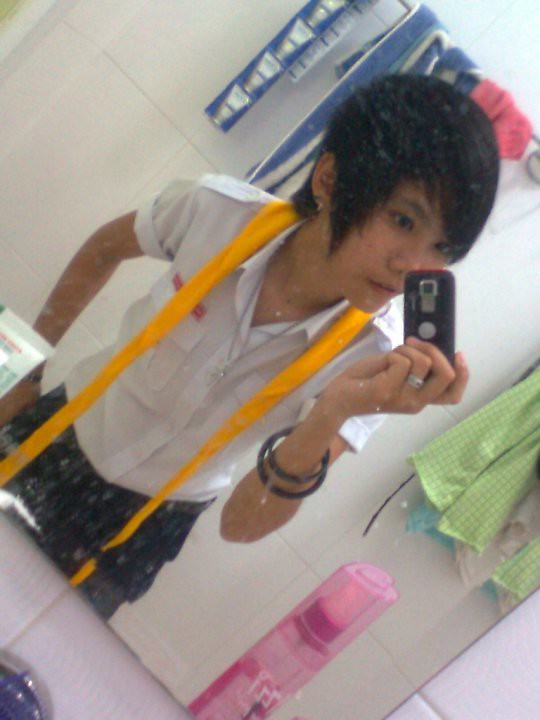In this photograph, an Asian woman is taking a selfie in a bathroom using an older model phone, possibly a Nokia. She has short, black hair styled with long sideburns and is looking at the phone screen rather than the mirror. She is wearing a short-sleeved, buttoned white collared shirt paired with black trousers. Around her neck hangs a long yellow lanyard that extends out of the frame. She also wears a necklace, two black bangles, and a silver ring on her left hand, which is holding the phone.

The bathroom setting includes a white tiled wall visible on both the left and right sides of the frame. In the background, blue and white towels are wrapped around a towel rack, and a small flannel is seen on the right. On the right-hand side of the bathroom counter, there is a transparent pink bottle with a lid resembling that of a hairspray bottle, which might be a spray or a water bottle. Additionally, the bottom part of light green clothing hanging from a hanger is visible.